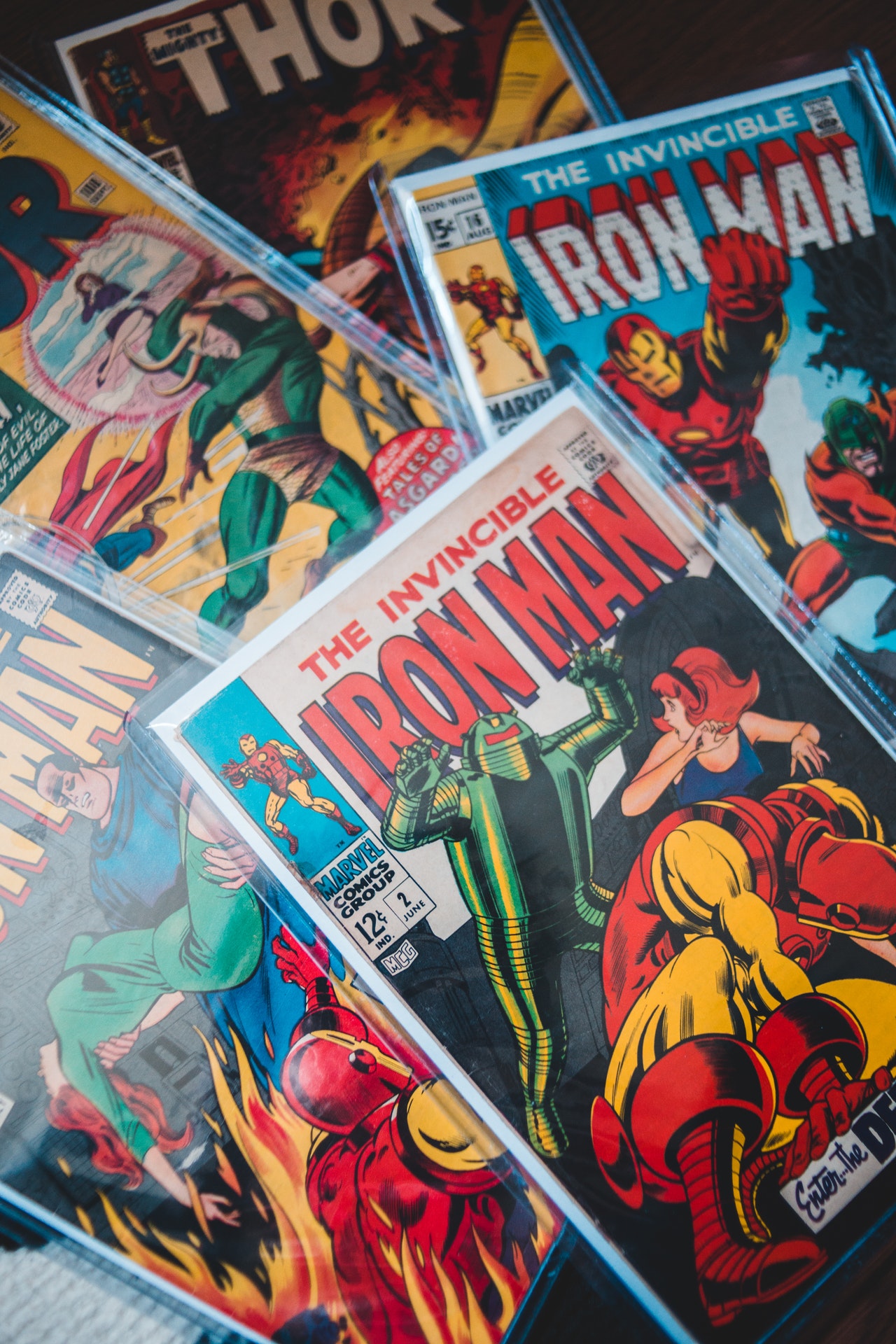This image showcases a vibrant collection of vintage superhero comic books, prominently featuring multiple covers of Iron Man and other characters. In the forefront, there's a dramatic scene from the Invisible Man series, where a terrified woman, dressed in a bulbous outfit, sits on a couch with a green robot monster stalking her; in front of her, a man appears to be kneeling. Above this, there’s an Invincible Iron Man cover with distinct red text, presenting Iron Man in action alongside a large creature. To the back, visible behind the piles of comics, is a classic Thor comic. Below this Thor cover is another one featuring Thor with a green-clad character. On the lower left side under the first Iron Man, another cover shows Iron Man heroically carrying an unconscious woman in a tight green suit. Overall, the comics exhibit a nostalgic, old-school aesthetic, highlighted by their vintage price tags of 12 and 15 cents, and colorful illustrations of Iron Man in various dynamic poses, such as crouching, flying, and combating foes.